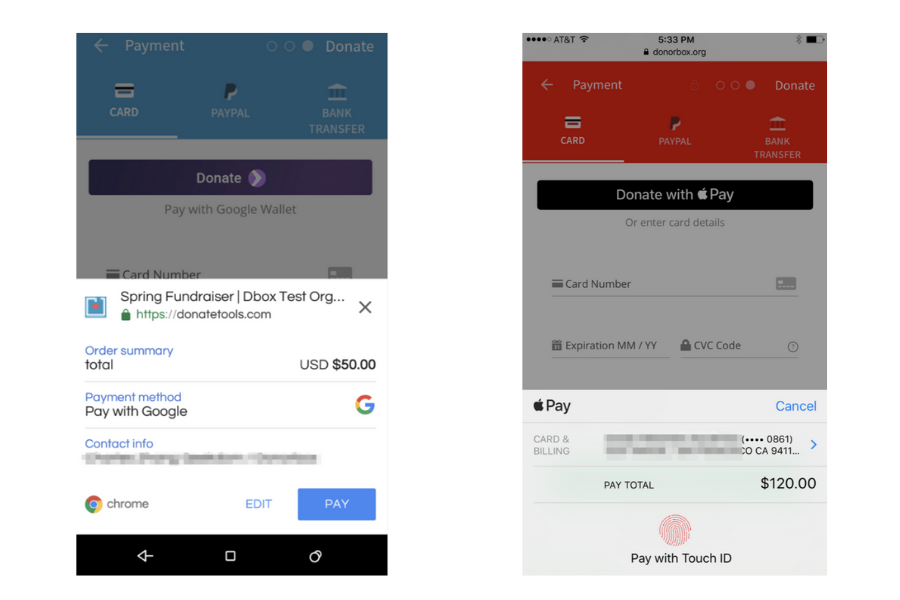The image is a composite of two screenshots taken from a cell phone, side by side, depicting various payment methods for donations.

On the left screenshot, the interface shows a payment section with options to pay via card, PayPal, or bank transfer. A prominent purple button labeled "Donate" is displayed, featuring a lavender circle with an arrow pointing to the right within it. The text beside the circle reads "Pay with Google Wallet." Below this, the details of a "Spring Fundraiser" are mentioned, hosted on DonateTools.com. The order summary lists a total donation amount of USD $50, and the payment method is specified as Pay with Google Wallet. The contact information for privacy is blurred out.

The right screenshot shows a payment page on DonorBox.org. Similar to the left, it offers payment via card, PayPal, or bank transfer. It also includes options to "Donate with Apple Pay" or to enter card details directly. Users can input their payment information, and at the bottom, it shows a transaction option to pay using Touch ID through Apple Pay, with a total payment amount of $120.

These screenshots illustrate different online donation interfaces, providing various payment options and highlighting the simplicity and security of modern digital transaction methods.